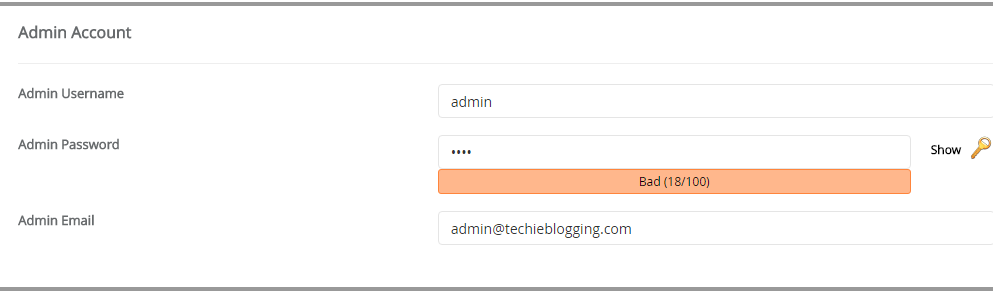The image features a white background with text and form elements. In the upper left corner, it reads "Admin Account" in black font. Below this, a thin horizontal line spans the width of the image. Underneath the line on the left side, there is a label that says "Admin Username." To the right of this label is a text box containing the word "admin."

Further down, there is another label that reads "Admin Password," accompanied by a text box to its right filled with four black dots, indicating that the password is hidden. Below these fields, a red box displays a warning message: "Bad 18 of 100." Directly beneath this red box, the label "Admin Email" appears, with a corresponding text box to its right that contains the email address "admin@techieblogging.com."